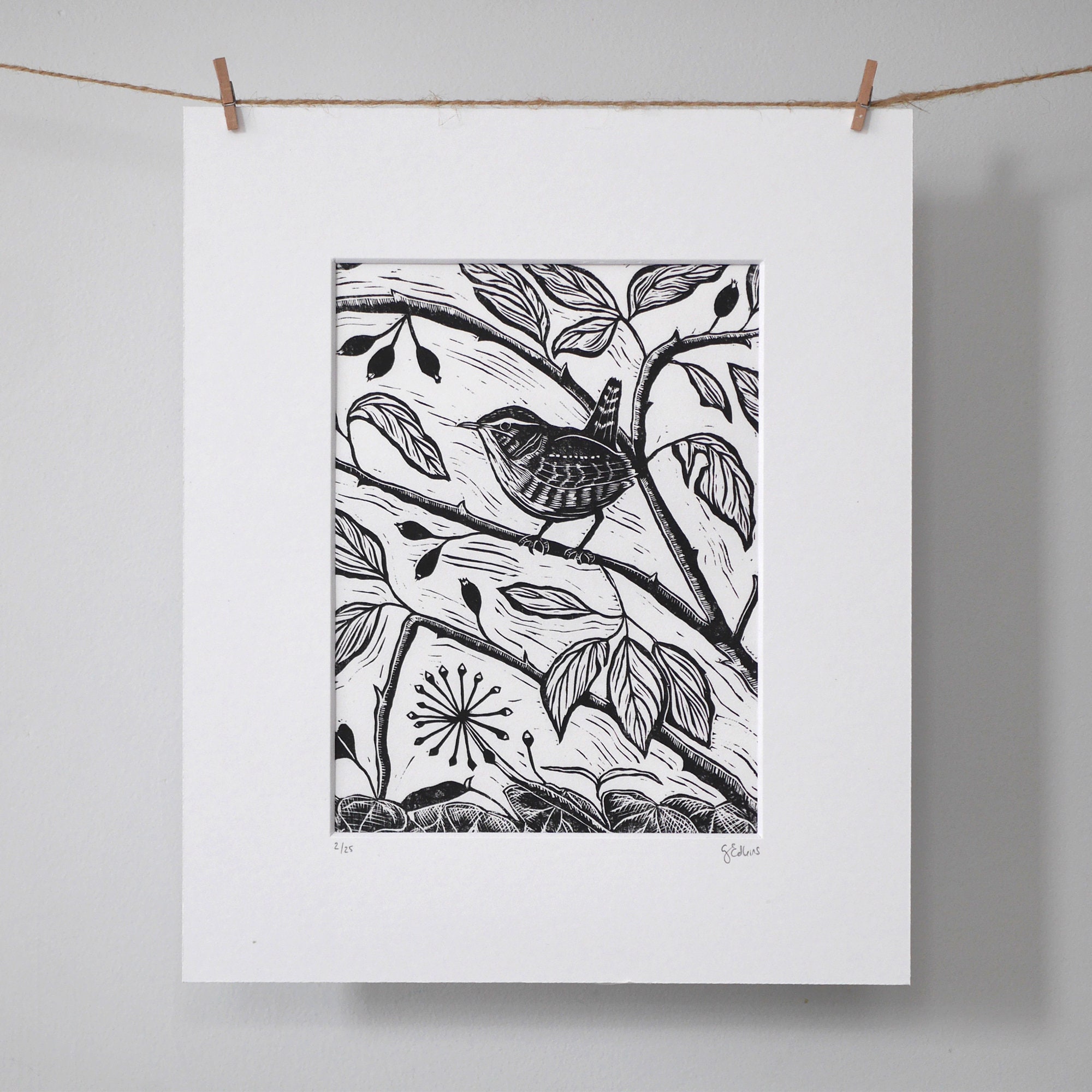The image showcases a detailed black and white sketch of a bird perched on a branch amidst leaves and flower buds. The setting gives a feeling of a natural outdoor scene captured artistically. Central to the composition, the bird, characterized by a darker upper body and lighter underside with distinct stripes, sits on the second branch from the top, looking to the left. Surrounding the bird are several branches, with a mix of detailed leaves and a prominently blooming flower at the bottom. The artwork is neatly matted with a white frame, adding to its presentation. It is displayed by being clipped at the top with two tan clothespins attached to a piece of twine that stretches across the top of the frame. In the bottom corners, there is an artist's signature on the right and a number - "2 out of 25" - indicating this piece is the second in a limited series of 25. The background features a simple gray wall, ensuring the focus remains on the intricate drawing.